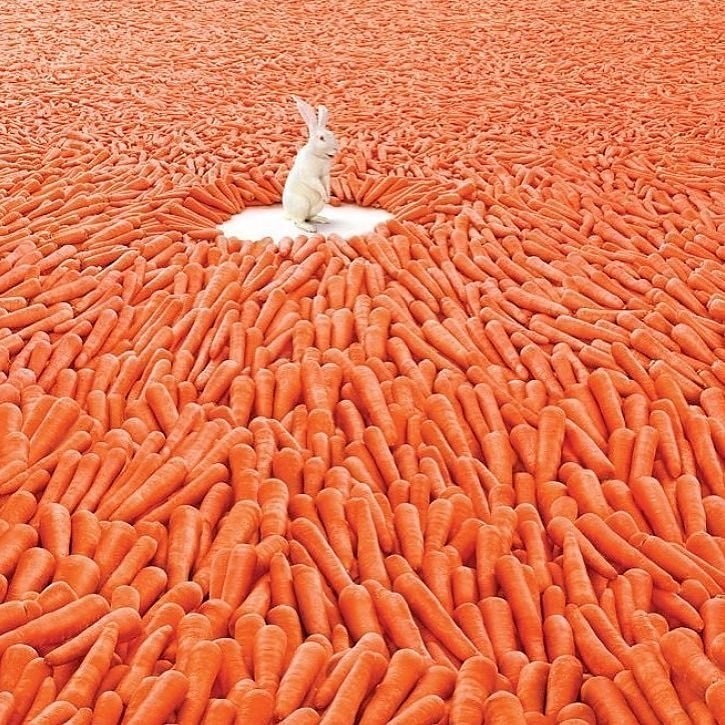This detailed color image likely created by AI, presents a whimsical scene featuring a white or light gray rabbit standing on its hind legs. Positioned slightly left of center in the upper portion of the frame, the rabbit is set on a stark white, circular platform, casting a slight shadow. The rabbit's ears are perked up and its face, shown in a three-quarter view facing to the right, displays a joyous, open-mouthed smile, as if in amazement. Surrounding this happy rabbit is an endless sea of vibrant, bright orange carrots, stretching from top to bottom and aligned to appear as if they're all pointing towards the rabbit. This surreal ocean of large, leafy-less carrots frames the image, with no text or additional elements to distract from the playful and fantastical scene.